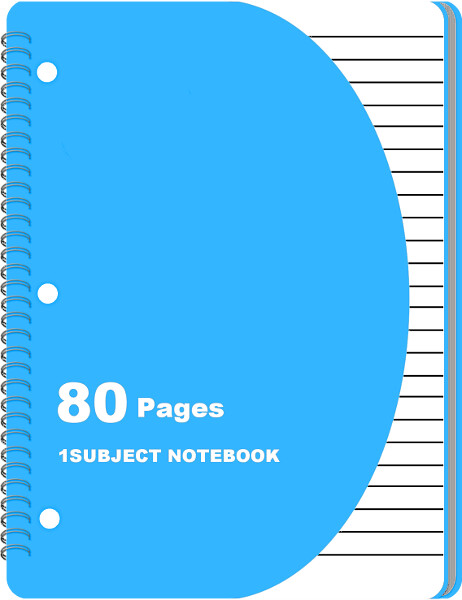This image is a detailed drawing of the front view of a one-subject notebook. The notebook is depicted in portrait mode with a light, sky-blue cover that has curved corners which bulge slightly outward before curving back in. On the left-hand side, dark gray metal spirals bind the notebook, clearly visible with three white dots representing the holes where the pages are held together. In white lettering on the lower left of the blue cover, it says "80 pages" followed by "One Subject Notebook." To the right side of the blue cover, partially visible, is a depiction of a white notebook page with black horizontal lines and two prominent vertical lines—one blue and one gray—extending from top to bottom, indicating the lined ruling of the paper inside. Overall, the notebook’s cover and design elements are vividly detailed, showcasing both the exterior and a hint of the interior pages.